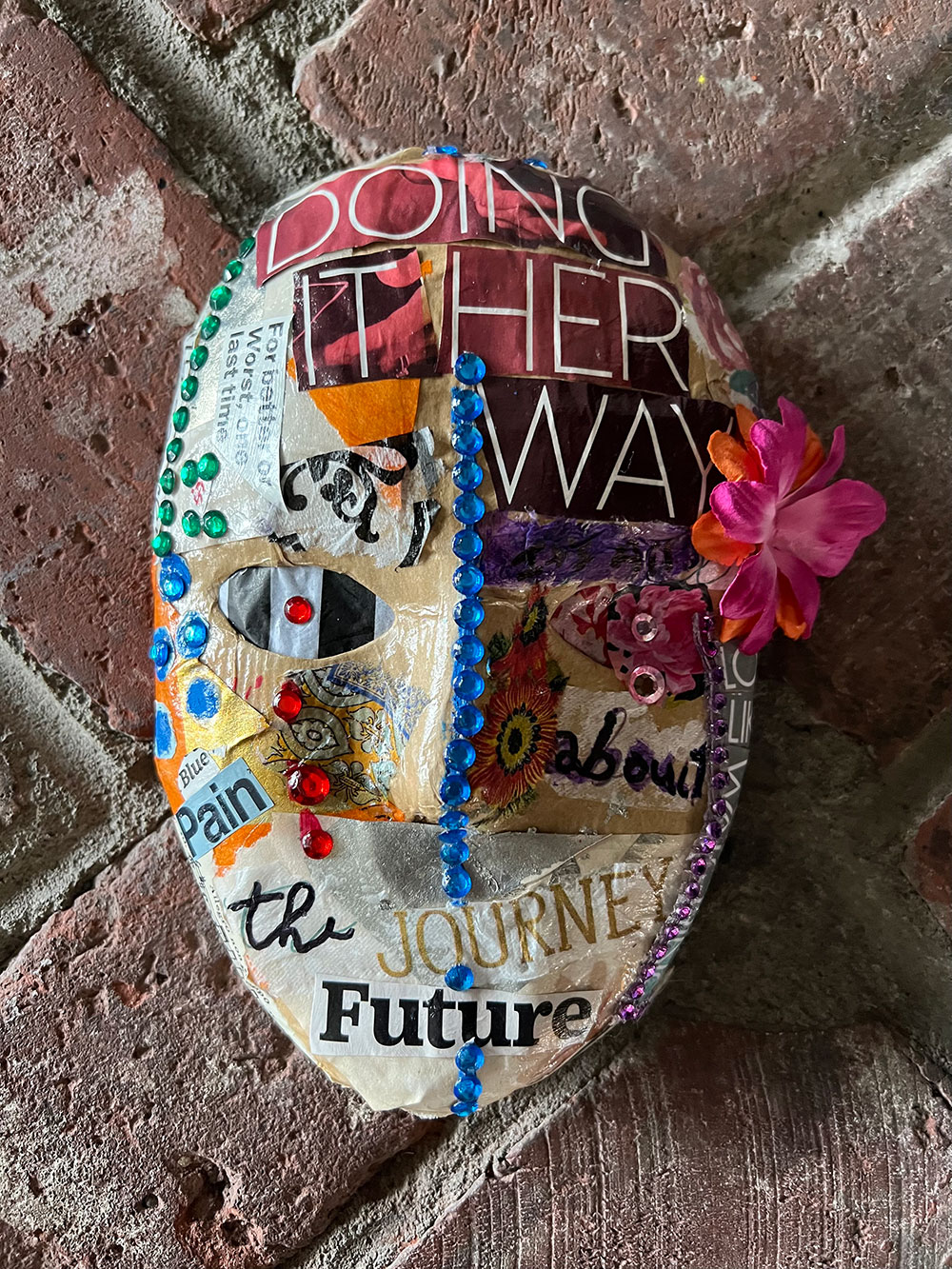This photograph captures a handmade, papier-mâché mask placed on a diagonal red brick surface. The mask, primarily beige, is intricately decorated with an array of magazine cuttings and colored glass beads, creating a mixed-media effect. Notably, a pink and orange rose adorns the left side (viewer's right) of the mask, accompanied by a variety of textual fragments such as "Doing it her way," "About," and "The journey future" prominently displayed across the face. 

The mask features a significant motif of blue beads running in a straight line from the forehead down to the chin. Complementing this, the left side of the mask is embellished with green glass beads. From the right eye socket, ruby-like beads cascade downwards, with one nestled centrally in the eye hole and three descending along the cheek, while the left side sports beads suggesting tears—either rubies or glass—arranged artistically down the cheek. Furthermore, decorating the left eye area are strokes of purple paint and smaller beads that extend down from the eye's corner.

Intriguingly, the mask lacks a mouth and has only one eye hole, focusing attention on the expressive, ornamented surface. Additional magazine cutouts, including "blue," "pain," and "last time," are meticulously placed across the mask, each characterized by unique fonts and colors, enhancing the overall artistic complexity. The base half of the mask transitions to a white-painted zone adorned with more textual elements, making this a compelling piece rich in visual and textual narratives.